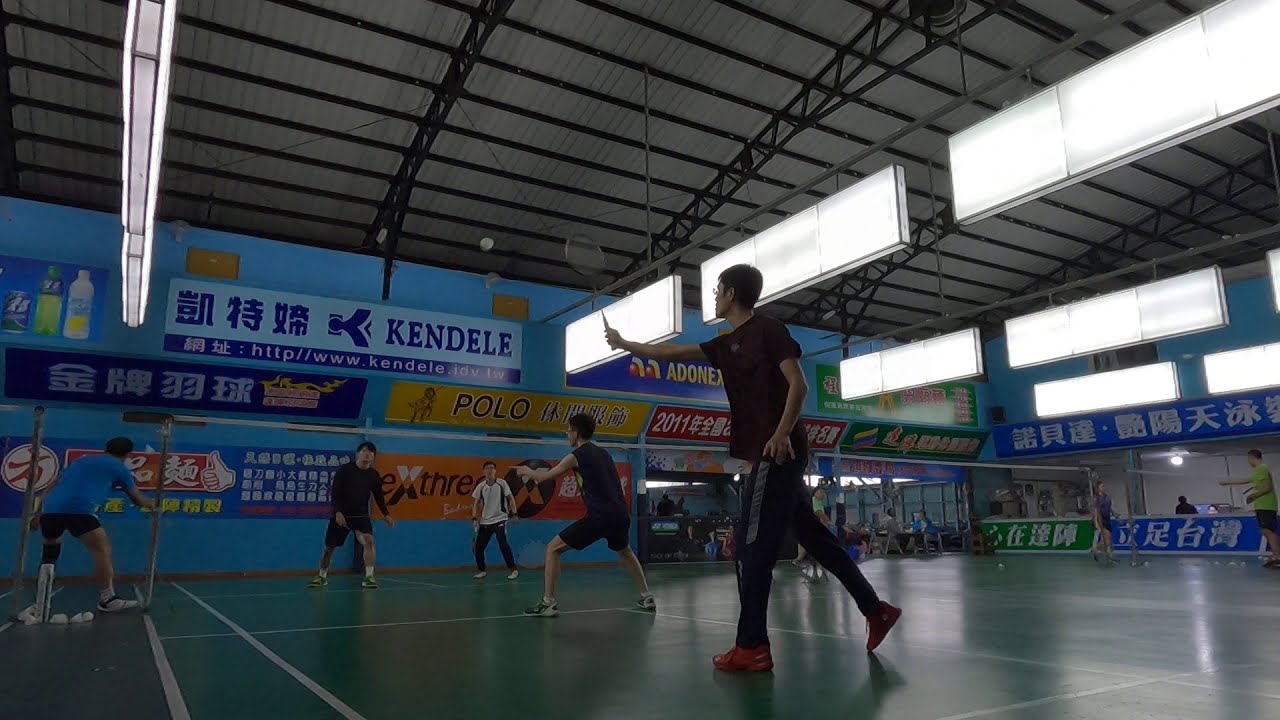The photograph captures an indoor badminton event taking place in a gymnasium equipped with metal framing and a ceiling supported by black beams. The ground is covered in a green surface marked with white lines that delineate three separate courts, each fitted with its own net. The scene showcases four players engaged in a match, two on each side, holding badminton rackets. A shuttlecock is visible in mid-air, emphasizing the action.

On the walls of the gym, several signboards and banners are displayed prominently. These feature a mix of Chinese characters and English text, with advertisements for various products such as "Polo" and "Kendall." The gym is illuminated by horizontal lights hanging from the ceiling, each spanning about 15 to 20 feet across. 

In the background, additional people can be seen, some of whom are seated at tables, suggesting a larger, possibly social or competitive event. The overall setting and details, including the presence of billboards and people standing or seated in the distance, evoke an energetic and communal atmosphere within the indoor space.